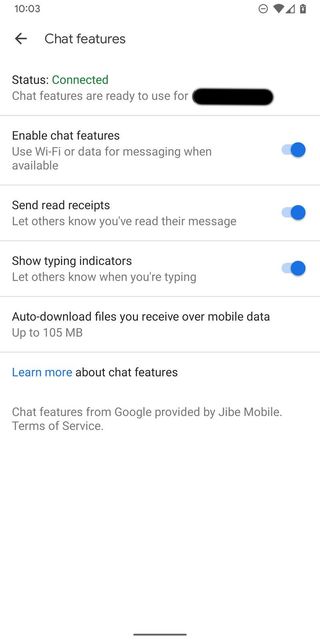Here is the refined and detailed caption for the image:

---

The image is a screenshot featuring a white background with predominantly gray text, accented by some green and blue fonts. At the top of the image, there is a status bar displaying the time as 10:03, along with several icons including a "Do Not Disturb" icon (a circle with a line through it), a Wi-Fi signal indicator, and a battery icon.

Beneath the status bar, there is a black back arrow labeled "Chat features". Below this header, the status of the chat features is indicated with the text "Status" followed by "Connected" in green. Underneath, in gray font, it reads "Chat features are ready to use for" followed by a section obscured by a black privacy blur.

The image continues with a section outlining options for chat features, each accompanied by a blue circular bullet point. The options are: 

- "Enable chat features"
- "Use Wi-Fi or data for messaging when available"
- "Send read receipts" (which allows others to know when their message has been read)
- "Show typing indicators" (which lets others know when the user is typing)

Further down, there is a subsection in black font detailing auto-download settings: "Auto-download files you receive over mobile data up to 105 MB", with a blue "Learn more" link adjacent to it. Following this is another black text item labeled "About chat features."

At the bottom of the image, gray text explains that chat features are provided by Google through Jibe Mobile, along with a link to the terms of service. Each section and option is separated by thin gray lines, making the image easy to read and navigate. Despite some pixelation, the text is bold and visually accessible, suitable for users including those with visual impairments.

---